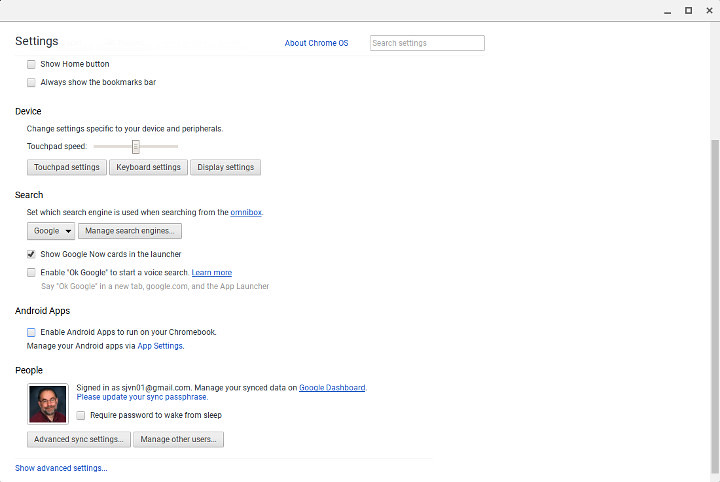This is a screenshot of the Google Chrome settings page. The overall settings interface appears somewhat blurred, but the left sidebar clearly displays the word "Settings." Centered in the middle of the page is the text "Chrome 06." Below the main "Settings" label, there are several options listed:

1. **Show Home Button**
2. **Always Show the Bookmarks Bar**
3. **Touchpad Speed** - Accompanied by a dial slider for adjustment.

At the bottom section of the screenshot, there are additional categories:
1. **People**
2. **Advanced Settings**
3. **Other Users**

In the top right corner, the 'X' button for closing the window is visible. The predominant color scheme of the settings page is white, interspersed with several blue hyperlinks. Each hyperlink consists of one or more words, presumably directing users to different settings or features within the browser.